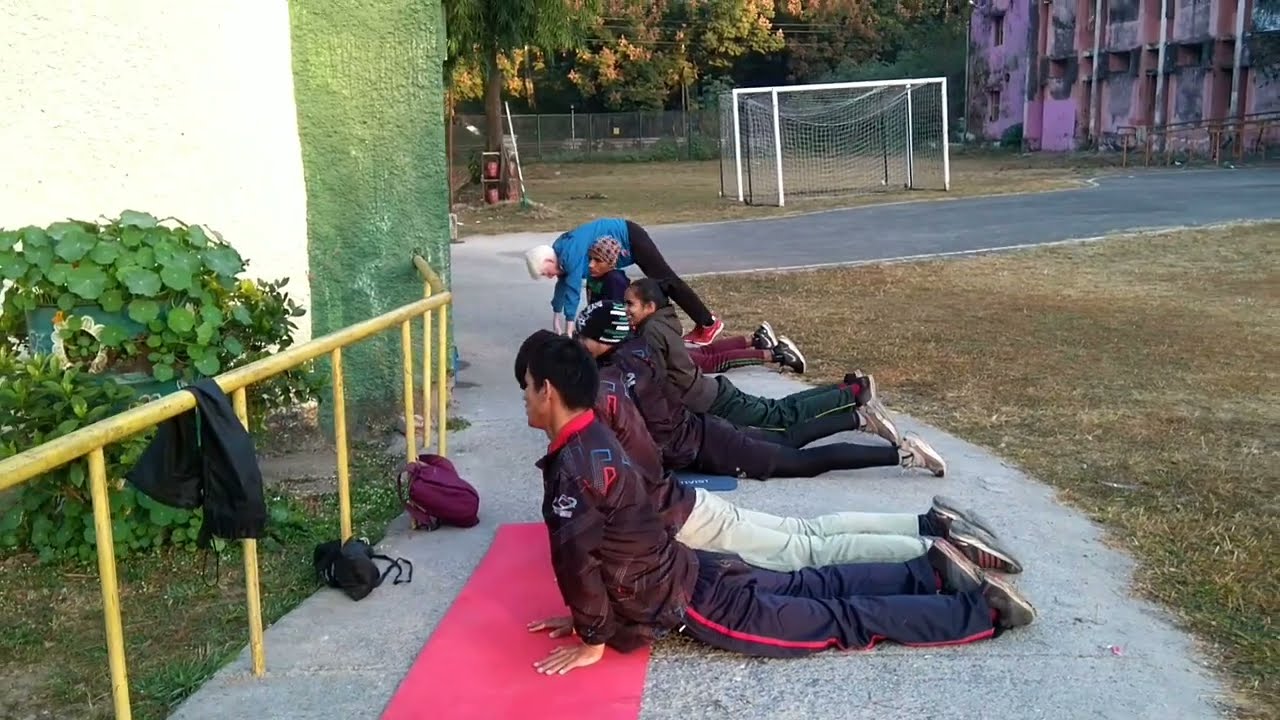In this detailed outdoor photograph, seven individuals are engaged in exercise poses on a sidewalk within a lush park setting. They are partially lying down and supporting themselves with their hands, adopting an interesting yoga-like position. Each person has a mat, with two using pink mats, and their backpacks and a jacket are casually placed nearby on the ground. The scene is set against a backdrop of greenery, featuring numerous trees and a fence enclosing the area right before the tree line. Dominating the right side of the image is a run-down pink and purple building. Also in view are power lines, a yellow railing in front of the exercisers, and a goal net, possibly for soccer, situated on the concrete. The individuals are scattered around the sidewalk, seemingly without a designated leader, absorbed in their routine. It is daytime, evidenced by the shadows cast on the ground, and the sky is clear, adding to the vibrant, relaxed atmosphere of the park setting.